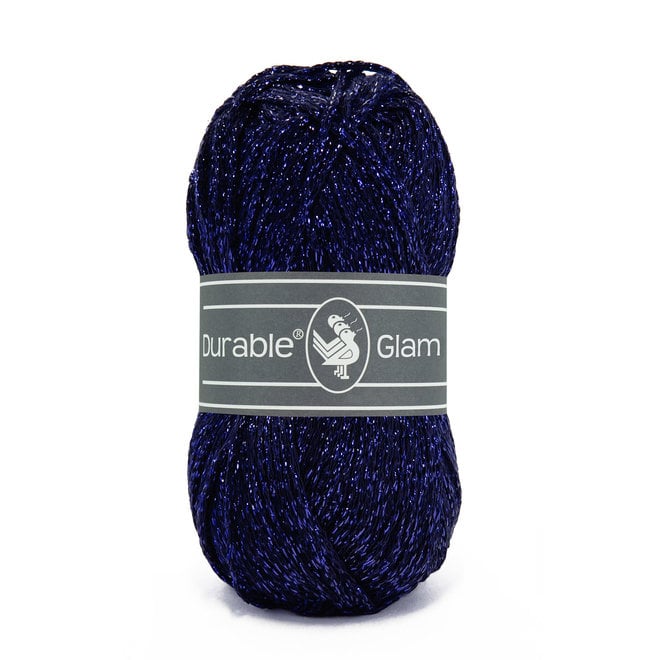This image features a close-up of a bundle of yarn, organized in a cylindrical shape and wrapped tightly in a paper or cardboard label. The yarn itself is a dark, midnight purple with sparkling white specks, resembling a starry night sky. The texture appears silky and shiny, reflecting light prominently. The label is grey with white horizontal lines and displays the text "Durable Glam" in basic white lettering. At the center of the label, an oval-shaped logo depicts three simple-shaped birds, likely ducks, oriented towards the top right. The background of the image is completely white, drawing all attention to the detailed features of the yarn and its packaging.